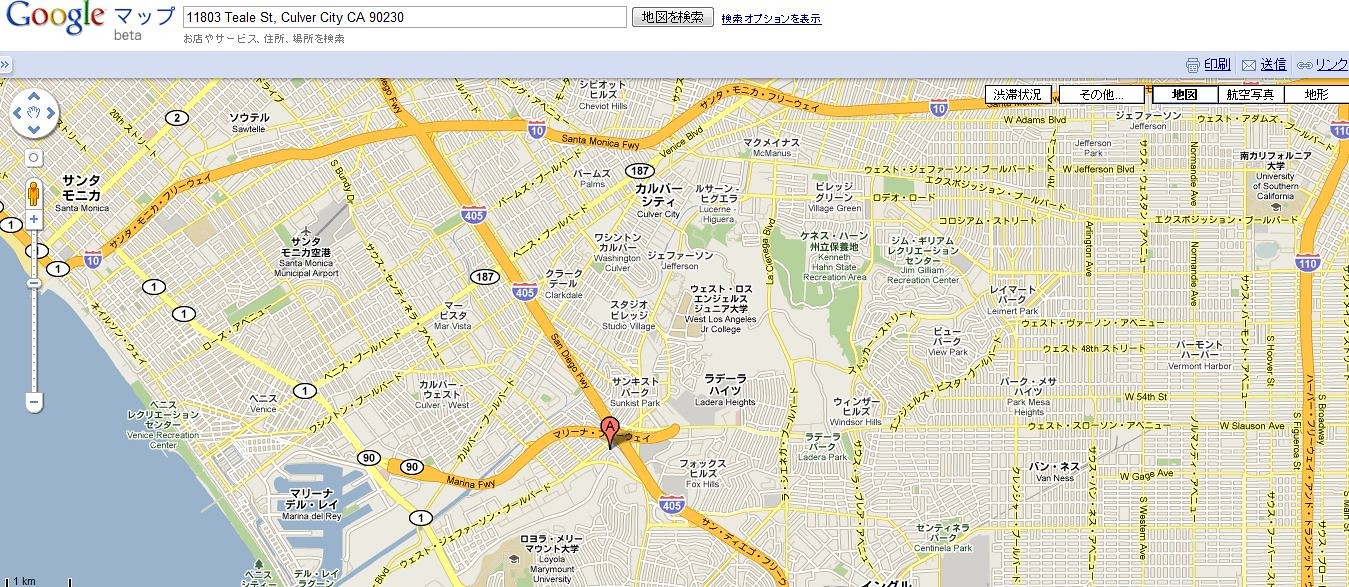This image is a screenshot of a Google Maps interface featuring a location in Carver City, CA. The map interface prominently displays the Google logo in the top left corner alongside a visible search bar with partially legible text starting with "11800." The text appears to specify an address in Carver City, CA. 

At the very top center of the image, there are characters likely from a language that uses symbols, possibly Japanese or Chinese. On the top right, there are four or five rectangular buttons, each inscribed with similar foreign language symbols.

The map itself is mostly white, with a distinct blue area situated towards the bottom middle to bottom left section, indicating a body of water - likely the coast of California. Several place names are scattered around the map; however, due to their small font size, they are quite difficult to read. Some names appear in English, presumably below corresponding foreign language names.

Additionally, four wavy yellow lines are present on the map, intersecting in seemingly random directions and positions, adding a layer of geographic information or possibly traffic data to the overall map view.